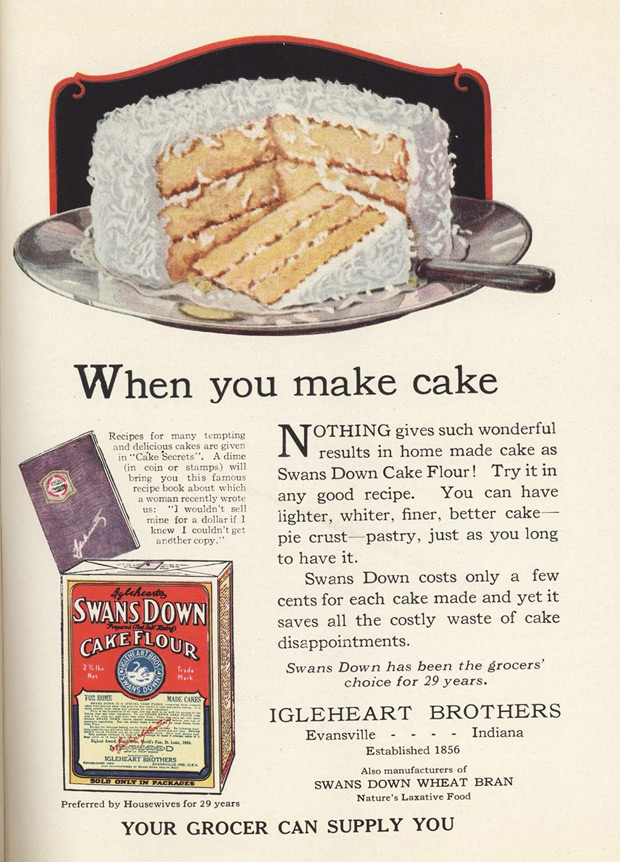This vintage advertisement, likely from the early 1900s, showcases Swans Down Cake Flour and features a striking image of a delectable coconut cake. The cake, presented on a clear glass plate, has a slice partially removed and resting in front of it. The cake reveals its soft, yellow interior contrasted by a rich chocolate icing topped with white coconut shavings. A silver knife is placed on the plate, suggesting the cake's recent cutting. Above this mouth-watering image, bold text declares, "When you make cake," emphasizing the superior results achieved with Swans Down Cake Flour. To the bottom left, there is an image of the iconic Swans Down Cake Flour box. The advertisement details the benefits of the flour, promising lighter, whiter, finer, and better cakes, pastries, and pie crusts. It assures readers of the product's cost-effectiveness, stating that it minimizes the risk of baking disappointments. The ad is attributed to the Iglehart Brothers of Evansville, Indiana, with a bottom line urging, "Your grocer can supply you."